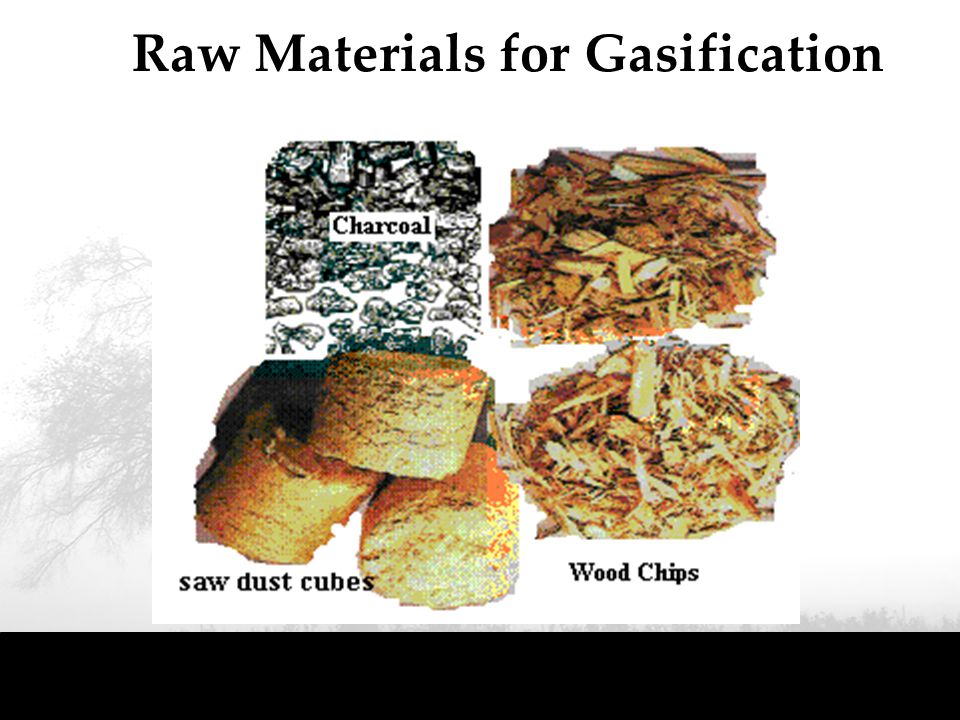The image is an informational slide titled "Raw Materials for Gasification," featuring four pictures arranged in a 2x2 grid on a white background with a black strip running along the bottom. The top left quadrant displays a black-and-white sketch of charcoal labeled "Charcoal," depicting a green and dark, rock-like appearance. Below this, in the bottom left quadrant, are "Sawdust Cubes," which resemble small oval hay bales or pieces of baguette. The right side of the grid is dedicated to "Wood Chips," with both the top and bottom right quadrants showing photographs of shredded, brown wood chips, although only the bottom right image includes a label. The background faintly hints at darker imagery, possibly reminiscent of trees or a smoky forest, enhancing the raw and natural theme of the materials presented.